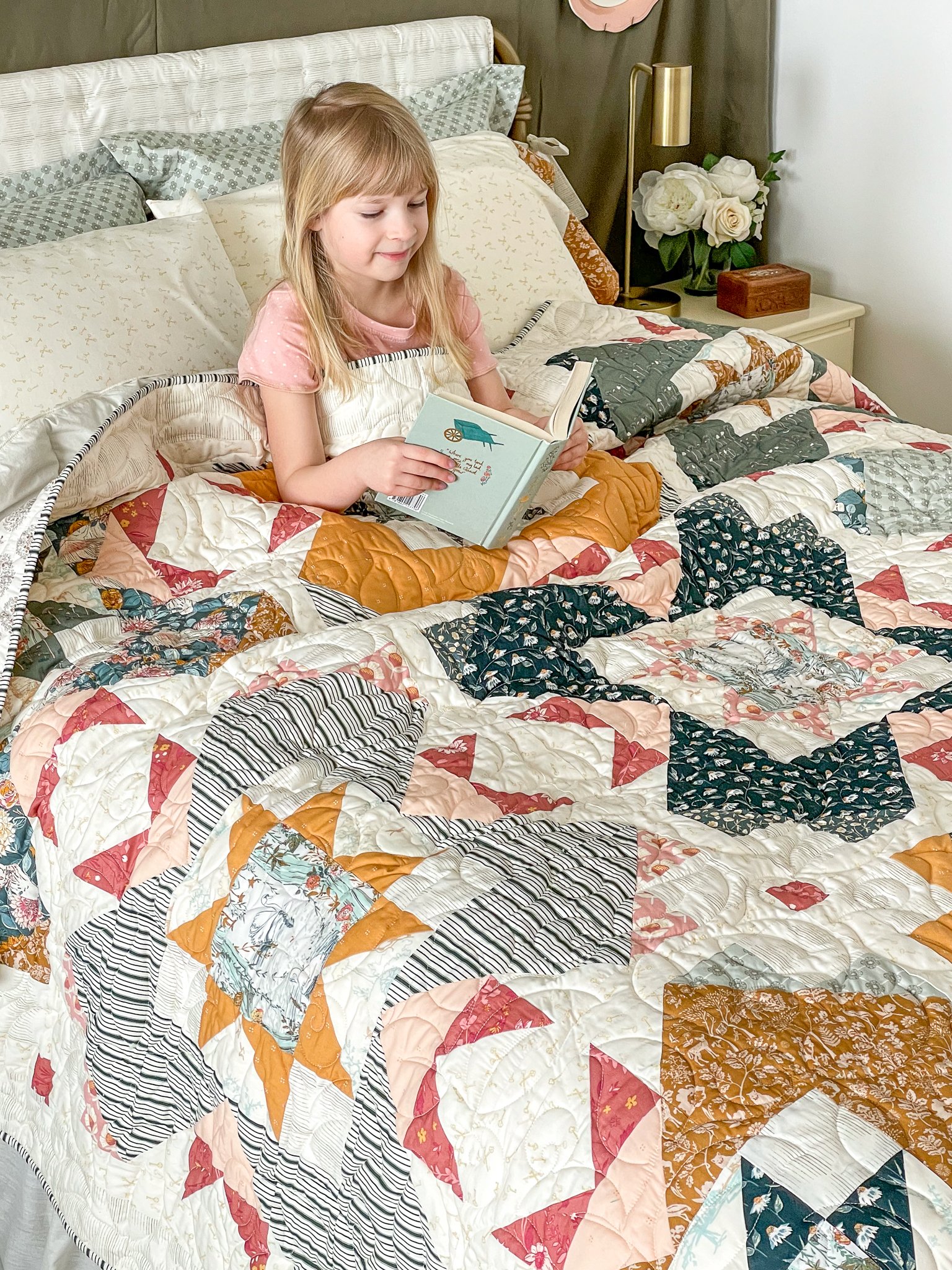In this indoor photo of a child's bedroom, a young blonde girl with medium-length straight hair and bangs is comfortably seated on her bed, engrossed in a blue book she is holding. She is dressed in a pink short-sleeve shirt and has very fair skin. The bed is adorned with a colorful quilted blanket featuring a variety of patches in different shades of greens, blues, whites, reds, and oranges, with floral prints and stripes interspersed. Behind her, four pillows are propped up—two are cream-colored, while the other two are green. The right side of the bed showcases a nightstand, which holds a bouquet of white roses, a small jewelry box, and a brass lamp. A dark green curtain or fabric is visible behind the bed, and the adjoining wall is a pristine white. The room is well-lit, highlighting the tidy and cozy ambiance.